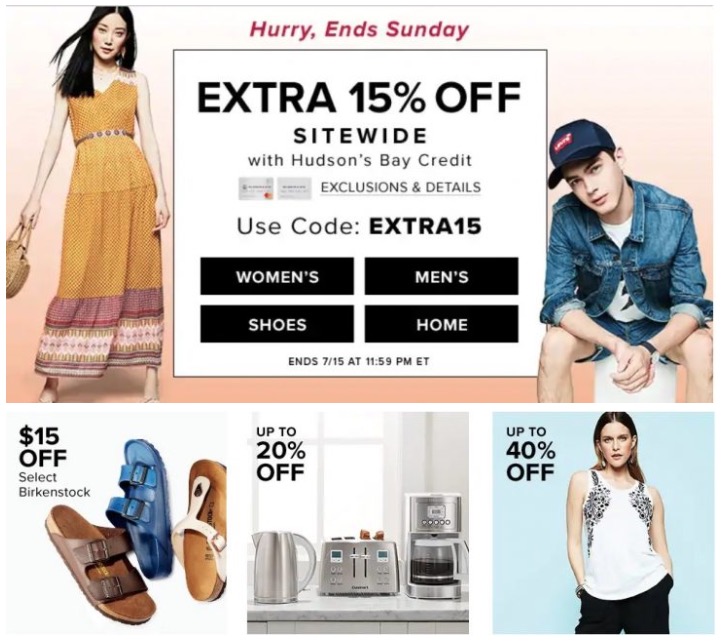An advertisement from Hudson's Bay showcases an exclusive "Hurry, Ends Sunday" promotion. Centrally highlighted in a square, the ad announces an extra 15% off site-wide with a Hudson's Bay credit card, mentioning exclusions and details. Shoppers are directed to use the code "EXTRA15." The offer spans across women's and men's apparel, shoes, and home categories, and is valid until July 15 at 11:59 p.m. Eastern Time. The advertisement features models dressed in various stylish outfits. 

Additionally, the bottom section highlights a $15 discount on select Birkenstocks, displaying three different styles, albeit only one shoe from each pair. Another segment promotes up to 20% off kitchen appliances, featuring an electric tea kettle, a toaster, and a coffee machine. Lastly, the ad boasts up to 40% off on select apparel, exemplified by a young Caucasian girl wearing a white t-shirt or tank top adorned with silver sequins, paired with black pants.